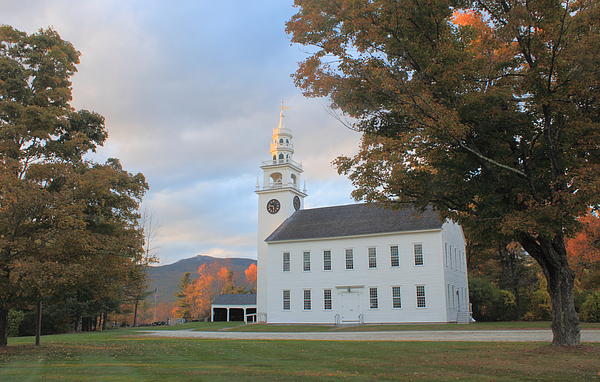This photograph showcases an elegant, rural church set against a picturesque countryside backdrop. The church is a two-story, white-painted structure featuring a triangular gray roof and a simple entrance with double white doors. The façade is adorned with two rows of windows—seven on the second story and six on the first, with three flanking either side of the main door. To the left of the church stands an impressive tower, combining elements of both a clock tower and a bell tower, crowned by a large white cross. A black clock face is visible on one side of the tower.

In the foreground lies a short green grass field, adding to the serene rural charm. A gray roadway runs from a garage adjacent to the church, leading off to the right side of the photograph. Complementing the scene are seasonal touches, with a combination of verdant greenery and hints of autumnal foliage. A large tree on the right and another on the left frame the church, while in the background, dark-colored mountains and orange-tinted fall trees hint at the seasonal transition. The sky above is light blue with grayish clouds, providing a gentle, calming canopy over the idyllic rural setting.